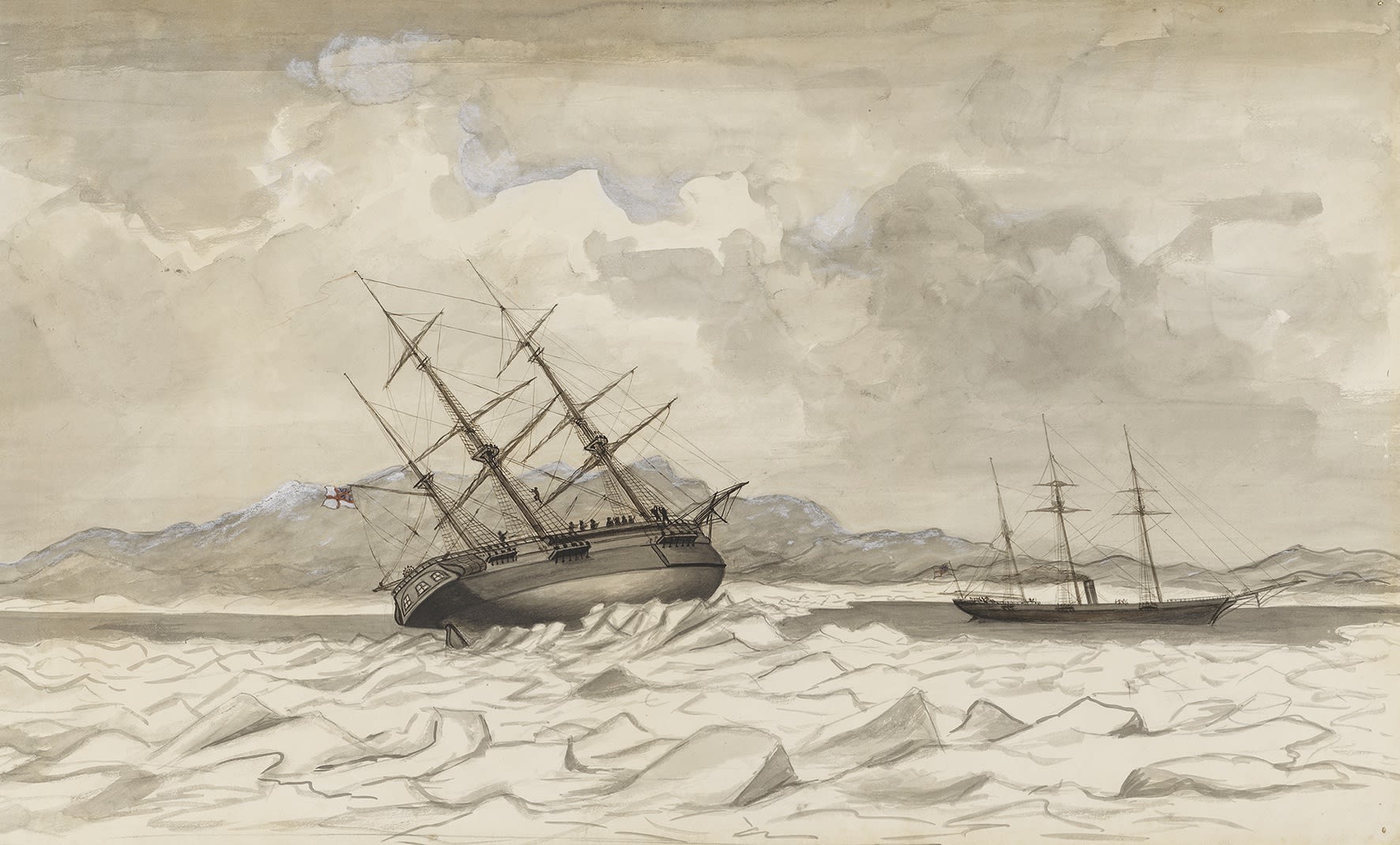The artwork portrays two old-time ships navigating stormy seas, evoking a sense of danger. The medium appears to be pencil and watercolor, characterized by muted grays and light beige tones. The ship on the left is dramatically tilted to the port side, seemingly on the verge of capsizing due to the large, rough waves. This ship, along with the upright one on the right, has three large masts without sails, indicating the severity of the storm. Dark gray clouds dominate the sky, enhancing the perilous atmosphere, while a mountainous island or hills loom in the background. The style of the piece suggests it may be from the 50s or 60s, or even earlier, consistent with the depicted ships' era.